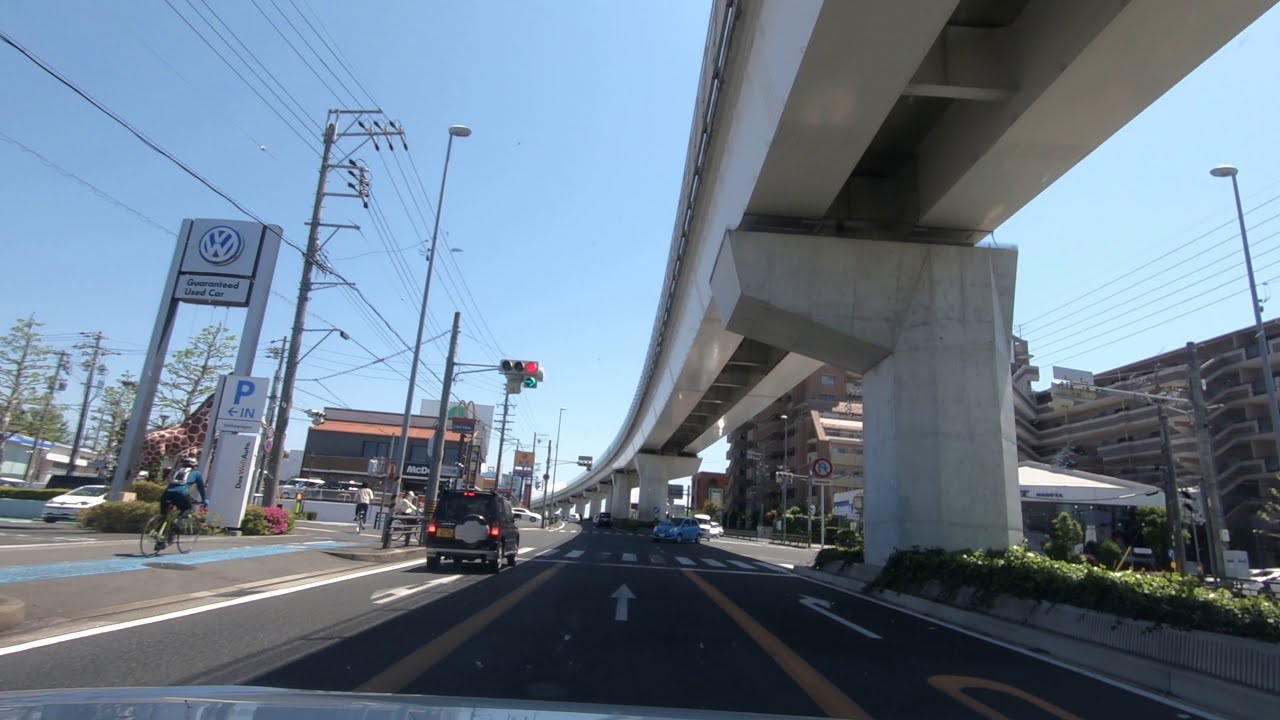The image captures the interior view of a car moving along an urban road. Above, the sky is a clear, light blue with no clouds in sight. The main focus is the white concrete overpass that stretches across the top of the road, casting a shadow on the three-lane street below. The lanes guide traffic with arrows indicating left, straight, and right turns. On the right side of the road, a residential high-rise features various patios, walkways, and stairs. Nearby, an electrical line and tall light posts add to the urban setting. Further along, a Volkswagen dealership, identifiable by its logo and "Guaranteed Used Car" sign, is visible to the left, with one white car parked inside and a man riding a bicycle in a designated bike lane. A dark SUV waits to turn left in the respective lane, while a blue car approaches from the opposite direction near a crosswalk at the road's end. Off to the horizon, a McDonald's and other buildings can be seen in the distance.